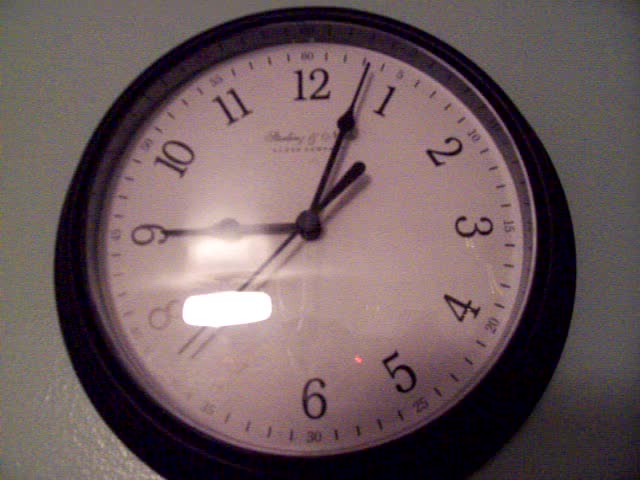This is a photograph of a standard wall clock with a classic design, prominently displayed against a gray backdrop. The clock features black hour, minute, and second hands, all clearly visible as they contrast sharply against the white face of the clock. The clock's outer rim is black, complementing the color of the hands. The current time displayed on the clock is 9:03, with the second hand positioned just two seconds before the eight. On the left side of the clock face, a reflection creates an elongated white rectangle, adding a touch of visual interest to the otherwise straightforward composition.